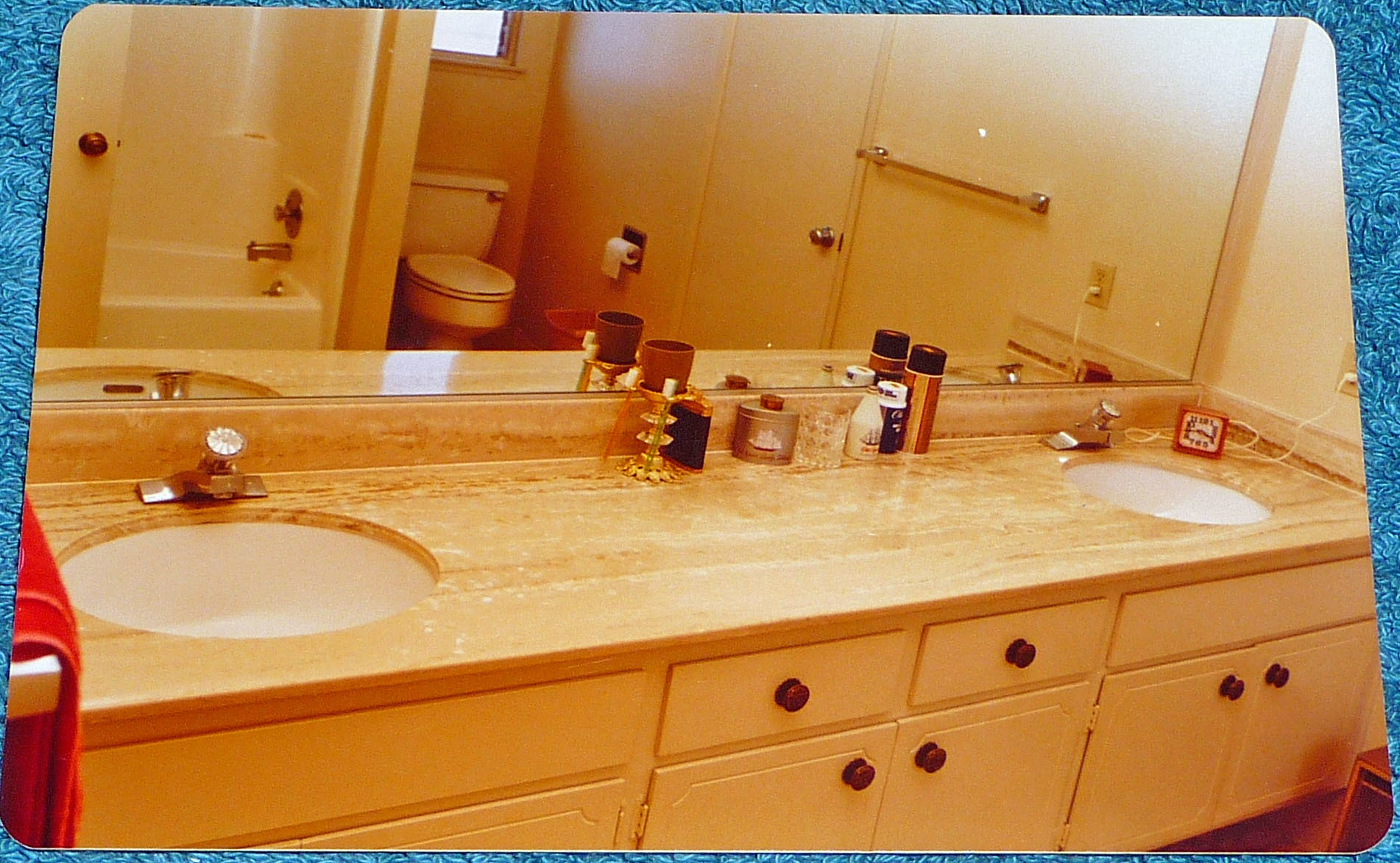In this detailed image of a bathroom, the focal point is a mirror set within a distinctive blue frame that resembles either feathers or a plush rug. Reflected in the mirror, the bathroom showcases a dual sink setup, providing ample counter space between the two washbasins. This area is utilized to hold various bathroom essentials such as candles, deodorant, and a small clock, contributing to a well-organized and personalized space. The background reveals additional bathroom fixtures including a toilet and a bathtub, partially visible through the reflection. The entire scene is bathed in a subtle yellow-brown filter, giving it a warm and somewhat vintage ambiance. The countertop material appears to be marble, enhancing the luxurious feel of the bathroom.